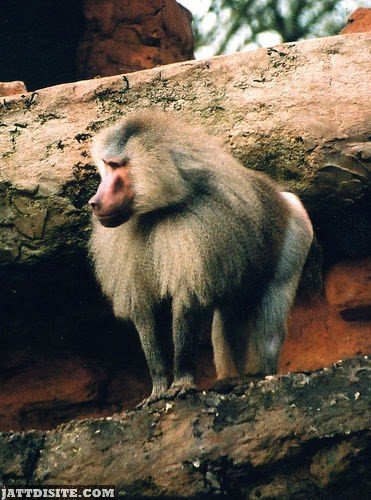In the image, there is a light-colored, furry monkey, possibly a baboon, standing on all fours on a rock ledge. The background features a blend of natural elements, including various shades of brown and red rocks, earthy terrain, and a blurred green tree or bush at the top. The scene is ambiguous, giving the impression that it could be either in a zoo or the wild. The monkey has a distinctive long snout and a pink face, and appears to be looking towards the left. In the bottom left corner of the image, there is text that reads "Jetisite.com" or possibly "JATTDISITE.com".